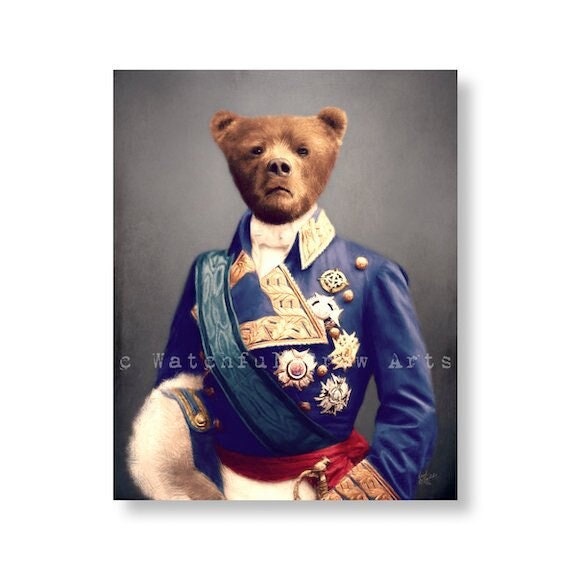The image is a detailed portrait painting of a brown bear with an upside-down triangle-shaped head, short ears, tiny black eyes, a round snout, and a serious expression with an upside-down smile. The bear is notably dressed in an elaborate and regal military uniform. This uniform consists of a blue long jacket with thick golden-embroidered collars and chest details, adorned with numerous medals and golden pins indicative of high rank. Notably, a red scarf or sash is draped around the bear's waist, complementing the silver buckle pieces on the jacket. To the right side of the bear's uniform, there appears to be a white material, possibly a cap belonging to the attire. The left side features a sword handle hanging from the body. The bear is set against a sophisticated studio-like grey gradient background. The image is marked with a faint watermark that reads "Watchful Paw Arts," and the artist's signature is visible at the bottom right corner.